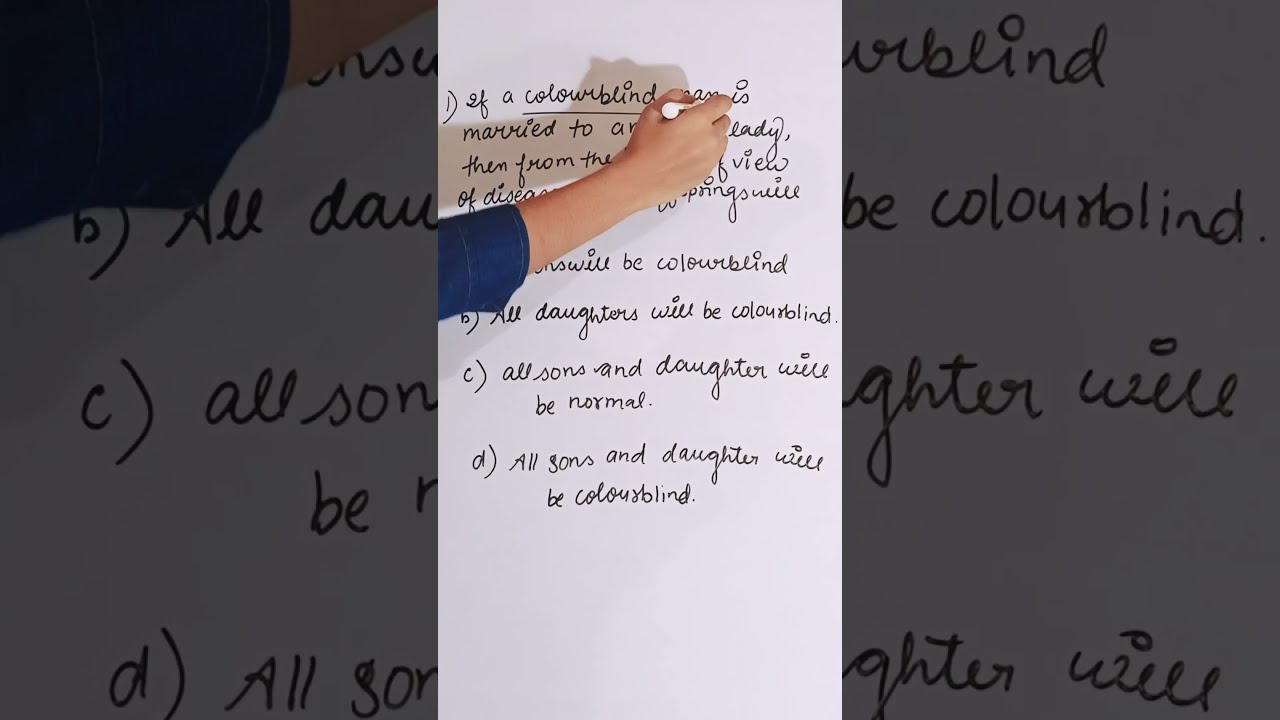In this horizontal rectangular image, we see a white piece of paper with text on it, positioned centrally against a background that appears to be an enlarged, partial view of the same text. Emerging from the left side of the image is a woman's arm clad in a blue elbow-length sleeve. The hand, belonging to a Caucasian person, holds a white marker and is partially obscuring the text on the paper, suggesting she is writing or underlining a list. The visible parts of the list include several genetic statements: "B) all daughters will be colorblind," "C) all sons and daughters will be normal," and "D) all sons and daughters will be colorblind." Despite some text being concealed by her hand, the context hints at a discussion of genetics, possibly in a classroom setting.